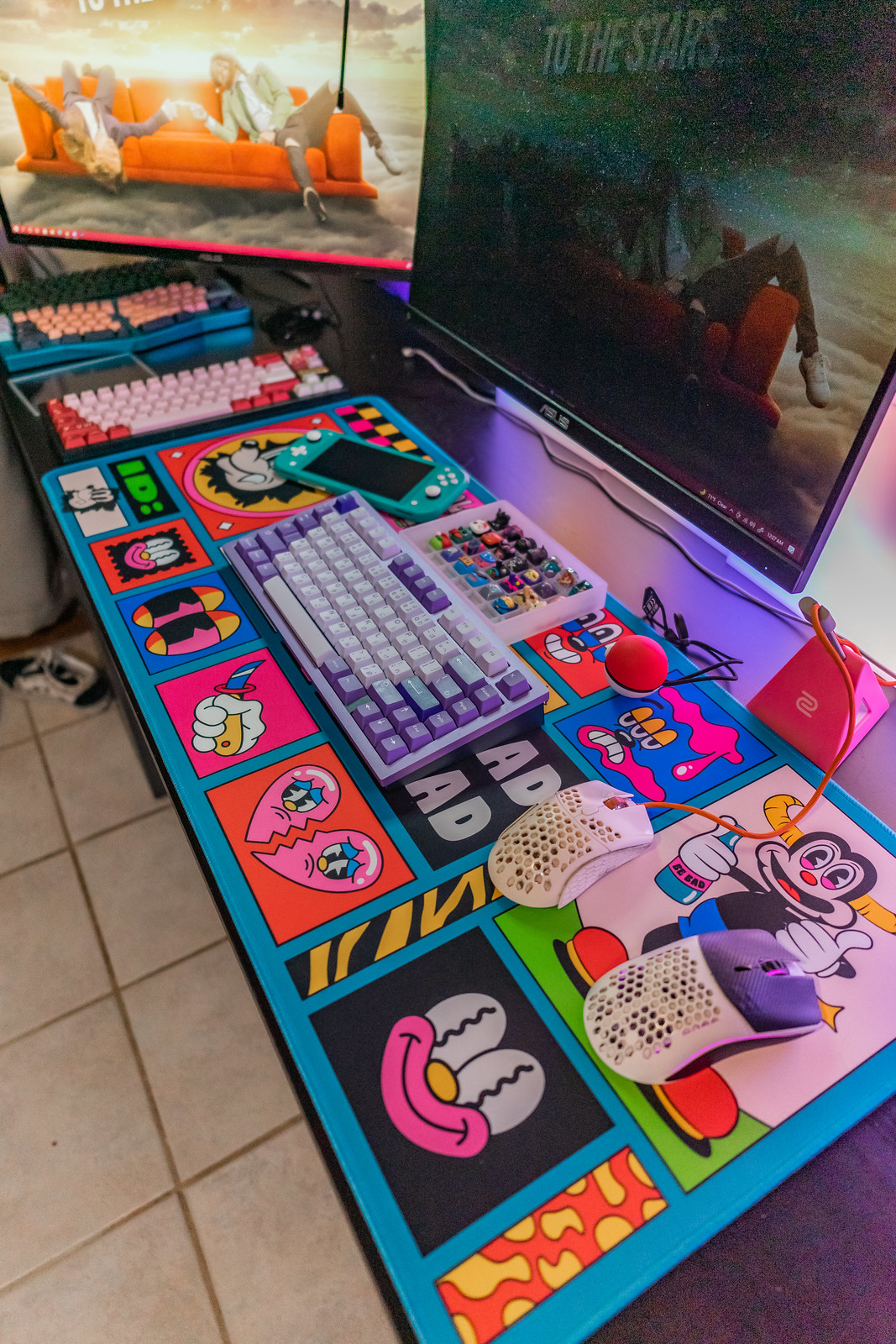This detailed image captures a vibrant and eclectic desktop setup on a beige-tiled floor. The desk is adorned with a colorful, graphic-designed desk cover featuring various cartoon images, including a broken heart with eyes, a wide pink smile with eyes and a yellow nose, and a cartoon monkey giving a thumbs up wearing big red shoes. 

At the center of the setup is a purple and white keyboard, paired with a matching purple and white mouse. Adjacent to this is another white mouse connected to a black monitor mounted above the desk. To the left, there's a second monitor angled to allow simultaneous viewing of both screens. Below these monitors are several additional keyboards: a pink and white one, a split blue one with white keys, and another keyboard featuring white keys with purple function keys.

The desk also holds a Nintendo Switch and a tackle-box-like container with small plastic figurines, hinting at the user's gaming enthusiasm. The entire arrangement is filled with bright, dynamic colors such as blues, pinks, oranges, and yellows, contributing to a playful and energetic workspace vibe.